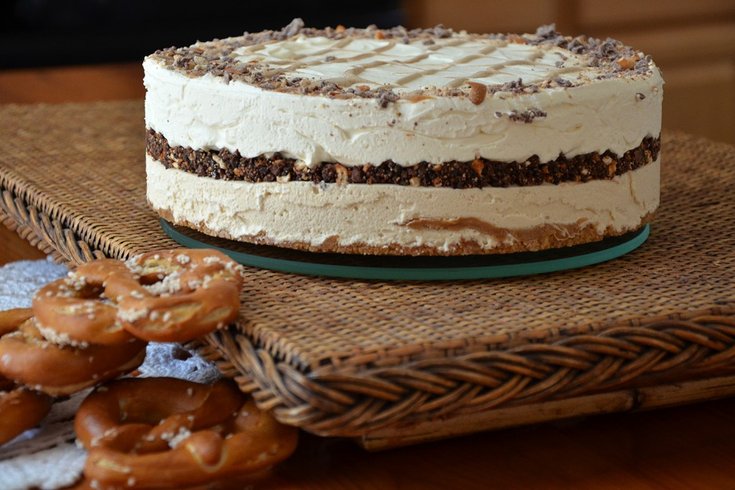The image is a well-composed, horizontal color photograph featuring an elegant, homemade-looking two-layer cake predominantly positioned slightly towards the top and right. The round cake is adorned with white frosting on the sides and top, encasing a middle layer of brown filling that resembles either chocolate or a cookie crumble like Oreo. Atop the cake, delicate garnishes, potentially chocolate pieces or nuts, are artfully sprinkled alongside decorative icing lines, adding subtle texture. The cake is placed on a turquoise and wooden-looking cake plate, which sits on a flat wicker basket. In the foreground, there are a few traditionally twisted, large brown pretzels with thick grains of salt, resting on a white doily-like napkin, creating a charming contrast to the central confectionery delight. The blurred foreground effectively draws focus to the cake, highlighting its intricate details and making it the center of attention in the photograph.